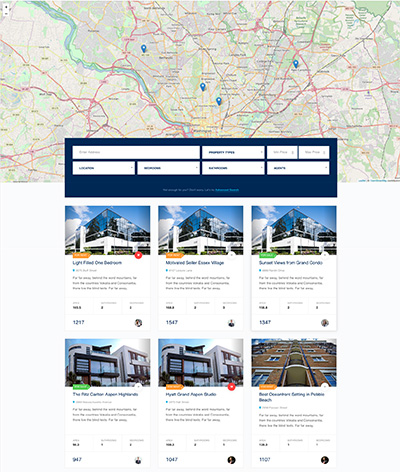This screenshot depicts a webpage from a travel website specializing in hotel accommodations. Though the resolution is limited, the general layout and content can be discerned. The upper section of the image features a map populated with pins indicating the locations of various hotels. Below the map, arranged horizontally, is a search bar that allows users to refine and filter their search criteria for accommodations. Further down, the main body of the page displays the search results: six thumbnail images of different hotels. Each hotel image is accompanied by details and pricing information, though the text is unreadable due to the low resolution. Despite the clarity issues, the structure of the page is evident, showcasing a map for hotel locations on top, a functional search bar in the middle, and visual hotel listings with brief descriptions and prices at the bottom.